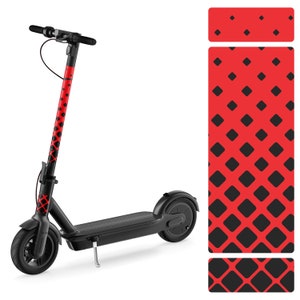This detailed product image showcases a sleek and minimalistic electric scooter designed with a striking red and black color scheme. The scooter features a thin, tall pole that is bright red and adorned with black diamond patterns, creating a bold visual contrast. The scooter's deck, along with its stand, wheels, and handlebars, is predominantly black, enhancing its clean and modern appearance. Notably, on the right side of the image, there is a flat mat or board displaying the same red and black diamond pattern as on the scooter, suggesting an emphasis on the cohesive design theme. This scooter, geared towards children, lacks a discernible brand name but includes functional elements like a small kickstand, and a visible mechanical tube near the handlebars, indicating its electric nature. The overall layout emphasizes simplicity and functionality in an attractive, eye-catching package.